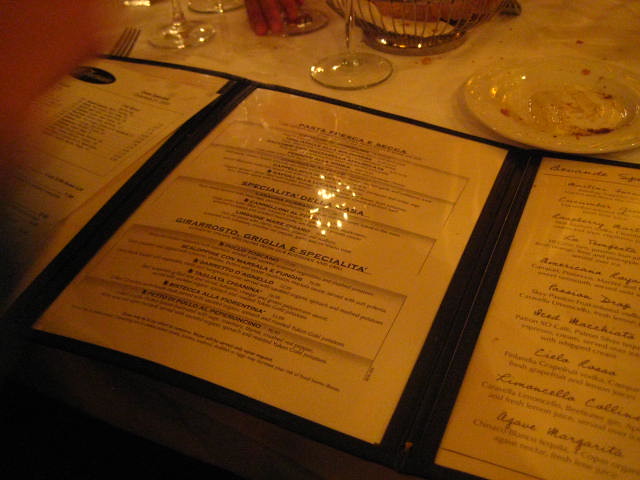An open tri-fold menu lies on a table adorned with a white tablecloth. The table showcases the remnants of a meal, with a messy plate stained with sauce and surrounded by crumbs. A silver wire basket, partially out of the frame, sits above the menu containing a white napkin and what appears to be a piece of brown bread. The stems of two wine glasses are visible just above the menu, adding a touch of elegance to the scene. The menu itself is difficult to read, possibly written in another language, with a significant glare from an overhead light source obscuring the text. In the background, a few fingers are caught in the frame, and the top left corner of the image is slightly obscured by a finger covering the lens. The lighting in the establishment is dim, casting subtle shadows and giving the photograph a moody atmosphere.